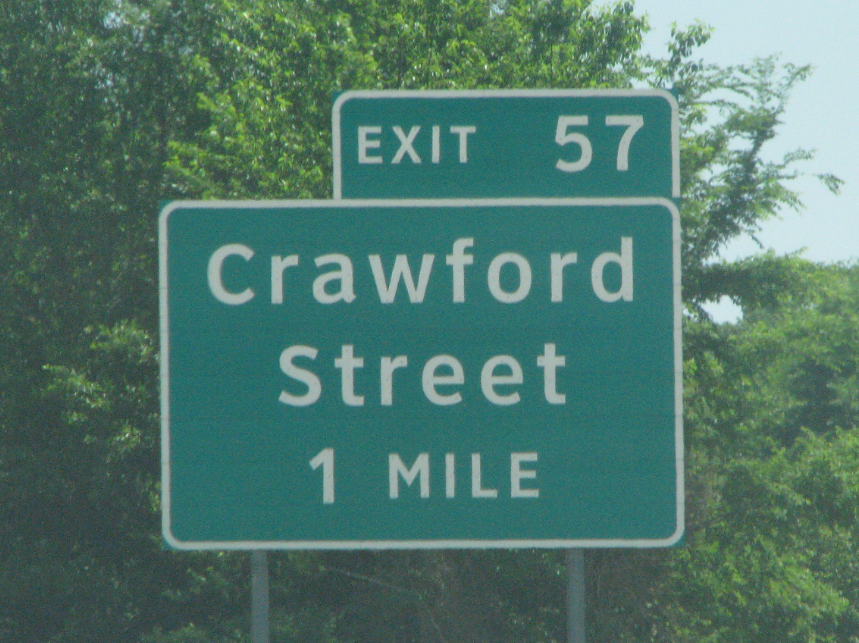This photograph features a prominent road sign set against a backdrop of tall, thick green trees with brown branches. The sign itself consists of two parts, both with a green background and a thin white border outlining the edges. The upper section of the sign reads "EXIT 57" in bold white text. Directly below, the main square section, approximately five inches in width, displays "Crawford Street" on the first line and "one mile" on the second line, also in white text. The sign is supported by two silver poles located on either side of the lower section. In the upper right corner of the image, a sliver of bluish-gray sky is visible, contributing to the overall daytime setting. The poles extend about two inches from the bottom, further anchoring the sign within the frame.